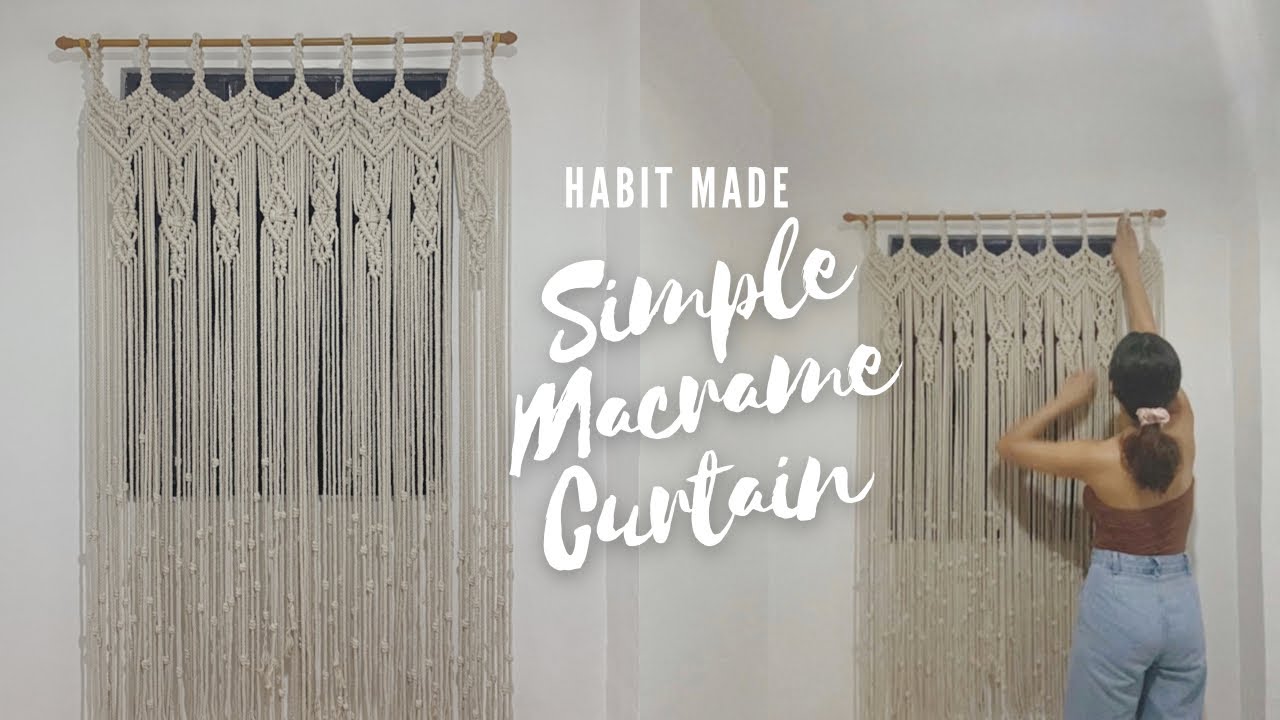The image features two side-by-side photographs of a room with a small white wall area displaying a doorway. The left photograph depicts a closed door adorned with a cream-colored macrame curtain, intricately designed and suspended from a brown rod. The curtain is made up of woven threads, forming a detailed and artistic pattern. In the right photograph, which mirrors the doorway from the left, a woman is seen standing in front of the curtain. She has her back to the camera, one hand reaching towards the top of the curtain rod and the other touching the curtain. The woman is dressed in a brown tank top, blue jeans, and has her hair tied back with a pink scrunchie. Between the two photographs, there's centered text that reads “HABIT MADE” in bold, white uppercase letters, and beneath it, in a lighter cursive font, “simple macrame curtain.”